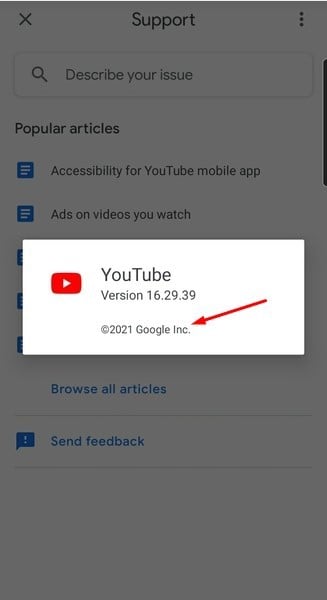A detailed caption for the image:

"Screenshot of the YouTube support page on a mobile device, overlaid with a pop-up highlighting 'YouTube version 16.29.39'. The background is dimmed to emphasize the pop-up, which is indicated by a red arrow. The pop-up includes a credit that reads 'Copyright 2021 Google Inc.' alongside the red Google Play button icon. Behind the pop-up, the support page is visible, displaying a header titled 'Support' and a search box with the prompt 'Describe your issue' next to a magnifying glass icon. Below, under the 'Popular Articles' section, there are links for 'Accessibility for your YouTube mobile app' and 'Ads on the videos you watch'. The bottom part of the screen, partially obscured by the pop-up, includes additional options such as 'Browse all articles' and 'Send feedback'."